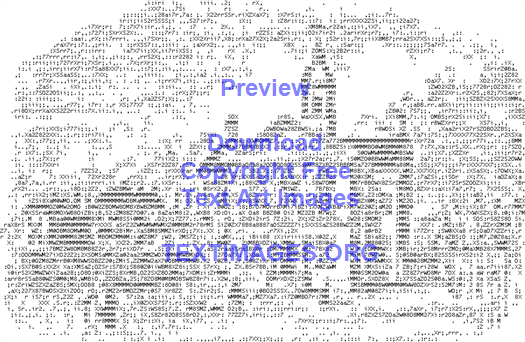The image features a detailed landscape created by an old dot matrix printer using a complex arrangement of black numbers, letters, and symbols on a white background. Central to the scene is a classical building resembling a church or cathedral, complete with tall peaks, a turret, windows, and surrounding trees, suggesting a natural setting. The artistic composition intricately simulates clouds in the sky, showcasing a high level of detail uncommon in simpler text art images. Overlaid in blue text is a watermark reading "preview, download, copyright-free text art images, textimages.org."